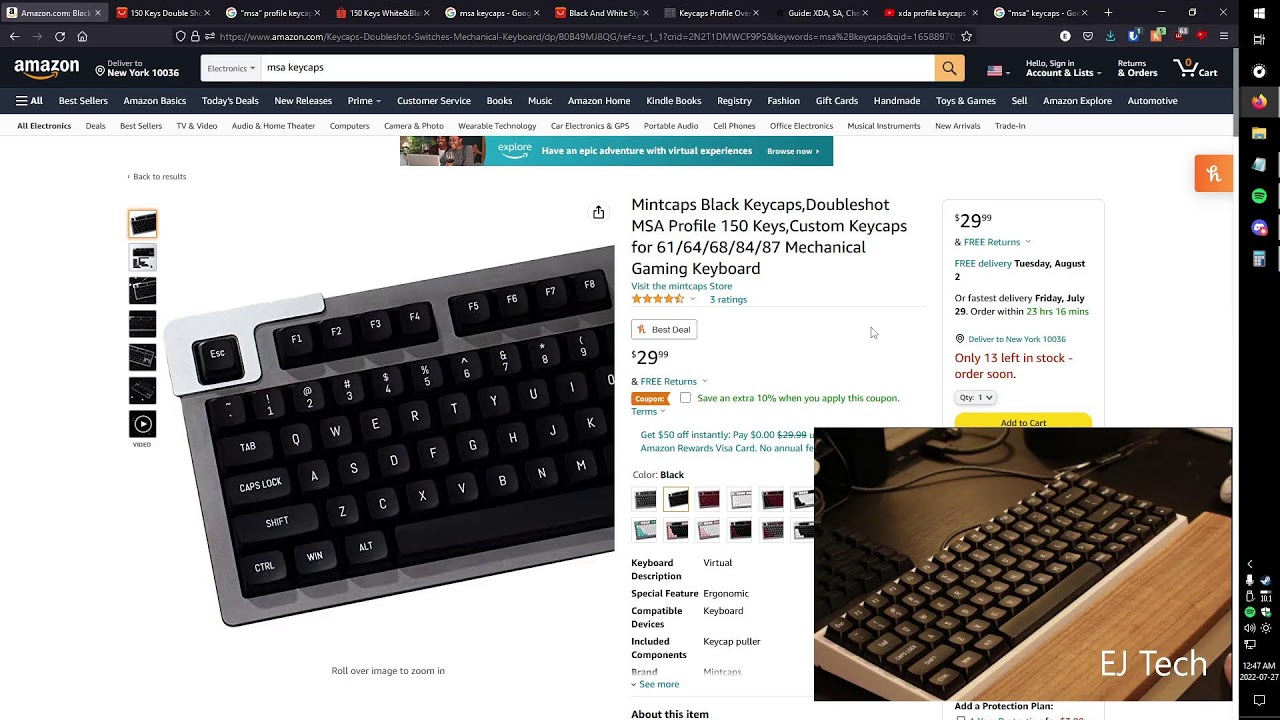This screenshot showcases an Amazon product page viewed within a Mozilla Firefox web browser window, which has a total of ten open tabs. The selected tab displays the Amazon website. The browser's interface features a black menu and border surrounding the webpage. The search bar on the Amazon page is set to the "Electronics" category, and the search term entered is "MSA keycaps."

The highlighted search result reveals part of a computer keyboard. The product is titled "Mint Caps Black Keycaps Double Shot MSA Profile 150 Keys Custom Keycaps for 61, 64, 68, 84, 87 Mechanical Gaming Keyboard." It is priced at $29.99 and has received three customer ratings, averaging at four and a half stars. In the lower right-hand corner of the screen, there is a pop-up image displaying the keyboard positioned on a desk.